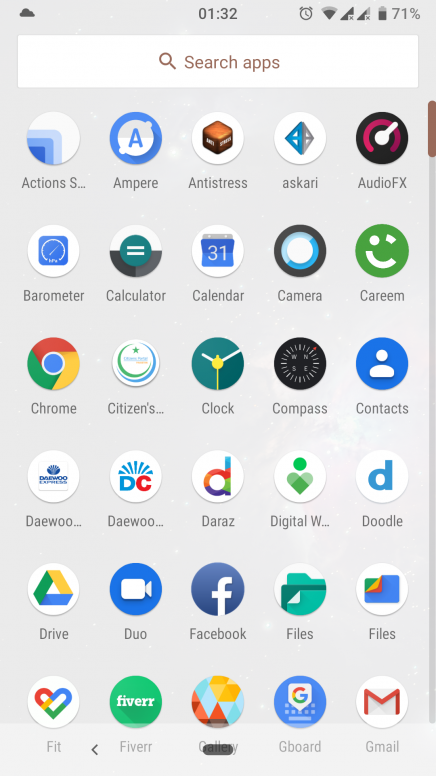The image appears to be a screenshot of an Android smartphone's app menu, shown in a grid format. In the top-right corner of the screen, there is a black cloud icon displaying "01 32", followed by icons for a clock, Wi-Fi signal, cellular signal, and a battery status indicating 71%. 

The header of the main screen features a search bar with the text "Search apps" in red, set against a white background, while the rest of the screen has a light gray backdrop. The apps are displayed in alphabetical order in rows:

1. **Actions S...**
2. **Ampere**
3. **Anti-stress**
4. **Ask Ari**
5. **Audio Effects**
6. **Barometer**
7. **Calculator**
8. **Calendar**
9. **Camera**
10. **Careem**
11. **Chrome**
12. **Citizens...**
13. **Clock**
14. **Compass**
15. **Contacts**
16. **Day Woo...** (two instances with different icons; the left one is blue, and the right one is lighter blue and red)
17. **Daraz**
18. **Digital W...**
19. **Doodle**
20. **Drive**
21. **Duo**
22. **Facebook**
23. **Files** (two instances; the left one with a teal icon, and the right one with Google colors - green, yellow, red, and blue)
24. **Fit**
25. **Fiverr**
26. **Gallery**
27. **Gboard**
28. **Gmail**

There is a scroll bar on the right side of the screen, slightly obscuring the last few app names.